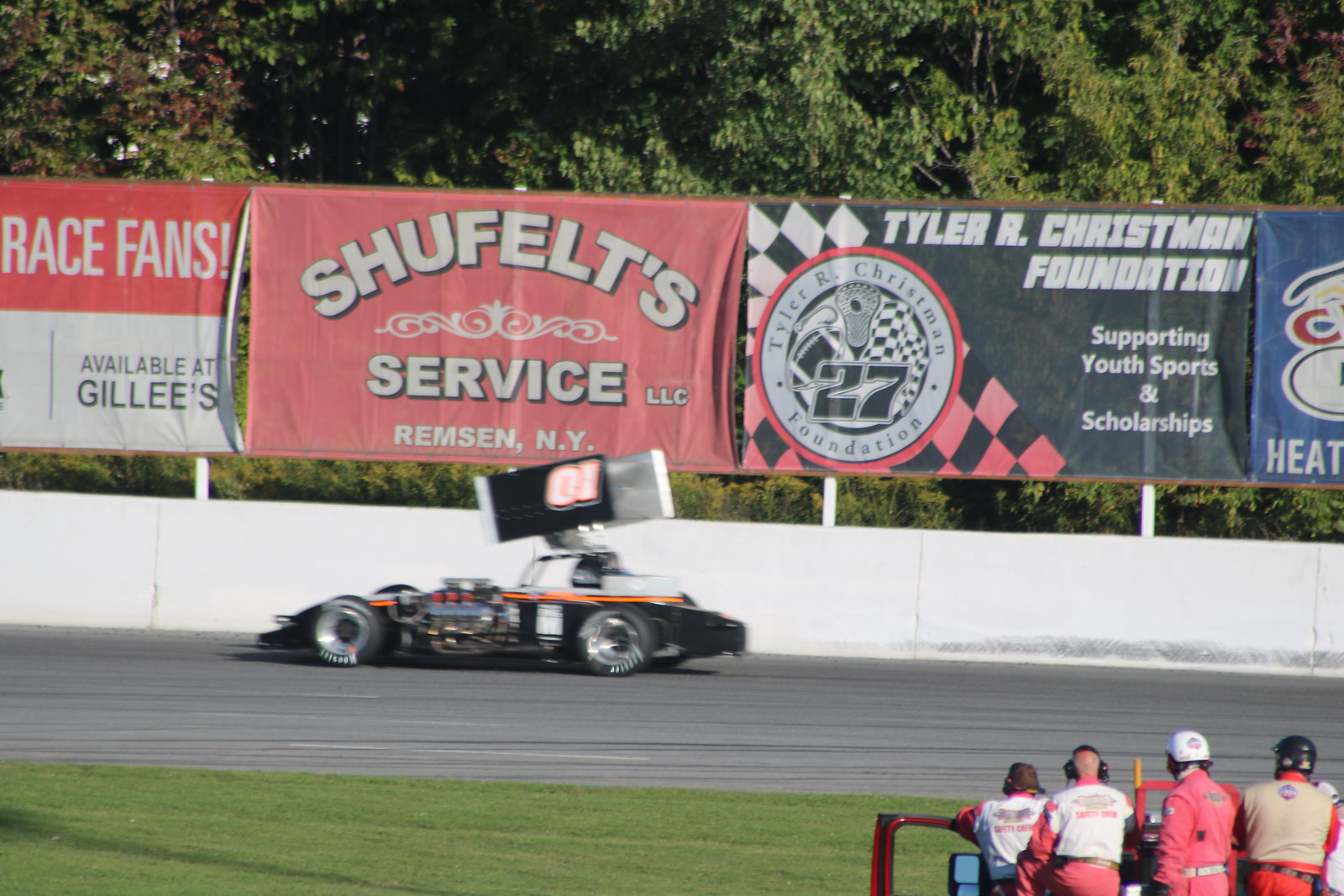This detailed photograph captures a dynamic scene at a racetrack during the daytime. Dominating the center-left of the image is a sleek, black race car with an eye-catching orange stripe. The car, low to the ground and winged at the top, appears to be in motion, contributing to a slight blur that emphasizes its speed. The racetrack's asphalt pavement stretches across the scene, with lush grass in the foreground.

To the lower right, a few onlookers, likely pit crew members dressed in red and some wearing helmets, attentively watch the race car. They stand out against a white half-wall that borders the track. Above the wall, a series of colorful advertisement banners catch the eye. The leftmost banner features red and white colors with the text "Race Fans" and "Available at Gillies." The next banner, set against a pink background, reads "Sheffield Services" followed by "Ransom, New York." Further to the right, another banner with a black background and white text promotes the "Tyler R. Christman Foundation." These details collectively evoke the excitement and vibrant atmosphere of a racing event.